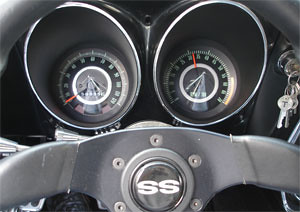The image captures the interior of an unidentified vehicle, focusing specifically on its dashboard and steering wheel. The dashboard features a sleek design adorned in chrome metal with accents of black and silver. Prominently positioned on the dashboard are two circular gauges: a speedometer and another measuring gauge, both housed in cup-like structures that resemble eyes when viewed closely. The steering wheel is detailed with five rivets encircling its center, providing a rugged touch. At the very center of the steering wheel, two white letters, "SS," stand out. In the upper right corner of the dashboard, the vehicle's ignition switch is visible with keys inserted. The composition of the image leaves the type of vehicle ambiguous, adding a layer of mystery to the scene.